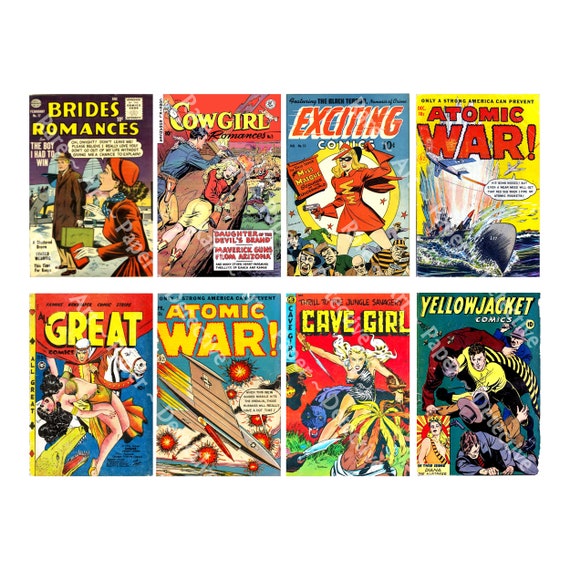This photograph features a vibrant grid of eight vintage comic book covers, arranged in two rows of four. These nostalgic covers, likely from the 1940s or 1950s, are adorned with bright reds and yellows that make them stand out. Each comic title is prominently displayed in bold, eye-catching letters at the top, with accompanying illustrations featuring a variety of characters and scenes.

Notable titles include "Yellow Jacket Comics," showcasing a superhero donned in a yellow shirt, black pants, and a black-and-yellow striped cape. Another cover, "Cave Girl," depicts a female protagonist akin to a caveman. "Brides Romances" presents an image of a man and a woman, emphasizing love and relationships. "Cowgirl" features a cowgirl and cowboy lying on rocks, capturing a Western theme. 

"Exciting Comics" highlights a woman in a red superhero outfit with a black mask. The intense scenes of "Atomic War" are represented by wartime imagery, including planes and battleships. The title "Just All Great" shows a man on horseback rescuing a scantily clad woman, a classic damsel-in-distress scenario. Another "Atomic War" cover focuses on a fighter jet in action.

Overall, the grid of comic book covers offers a window into the diverse and vivid storytelling of the mid-20th century, brought to life with dynamic colors and bold illustrations.